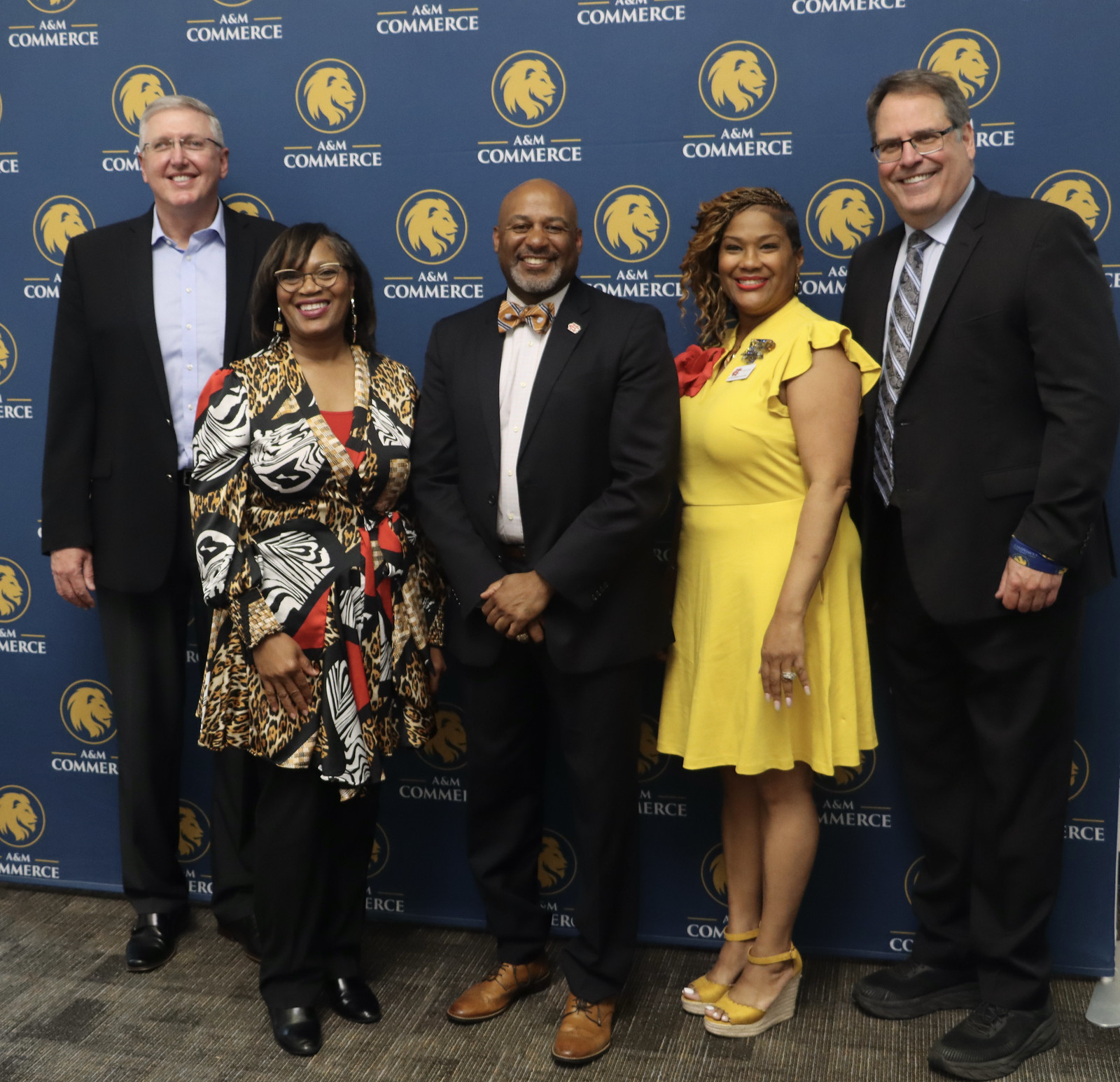In this detailed image, five elegantly dressed people are posing for a photo in front of a blue backdrop adorned with a repeating logo of a lion’s head in a gold circle and the text "A&M Commerce." Starting from the left, there is a white man with short grey hair and glasses, wearing a black suit and a blue shirt open at the neck, smiling warmly. Next to him stands an African American woman, around 40 to 45 years old, also with glasses, dressed in a colorful robe in gold, black, white, and red, with black pants and shoes. At the center is an African American man, bald with a grey beard, donning a black suit, a gold and brown bow tie, and brown shoes, with his hands crossed in front of him. To his right, there is another African American woman with brown hair, wearing a knee-length yellow dress, yellow and cork shoes, and a red rose pinned above her right breast. Finally, on the far right stands an overweight white man with glasses, dressed in a black suit and a striped blue tie, his left hand positioned at his waist. All five individuals are smiling and facing the camera, standing on a brown floor in front of the A&M Commerce banner, exemplifying a formal and joyous occasion.